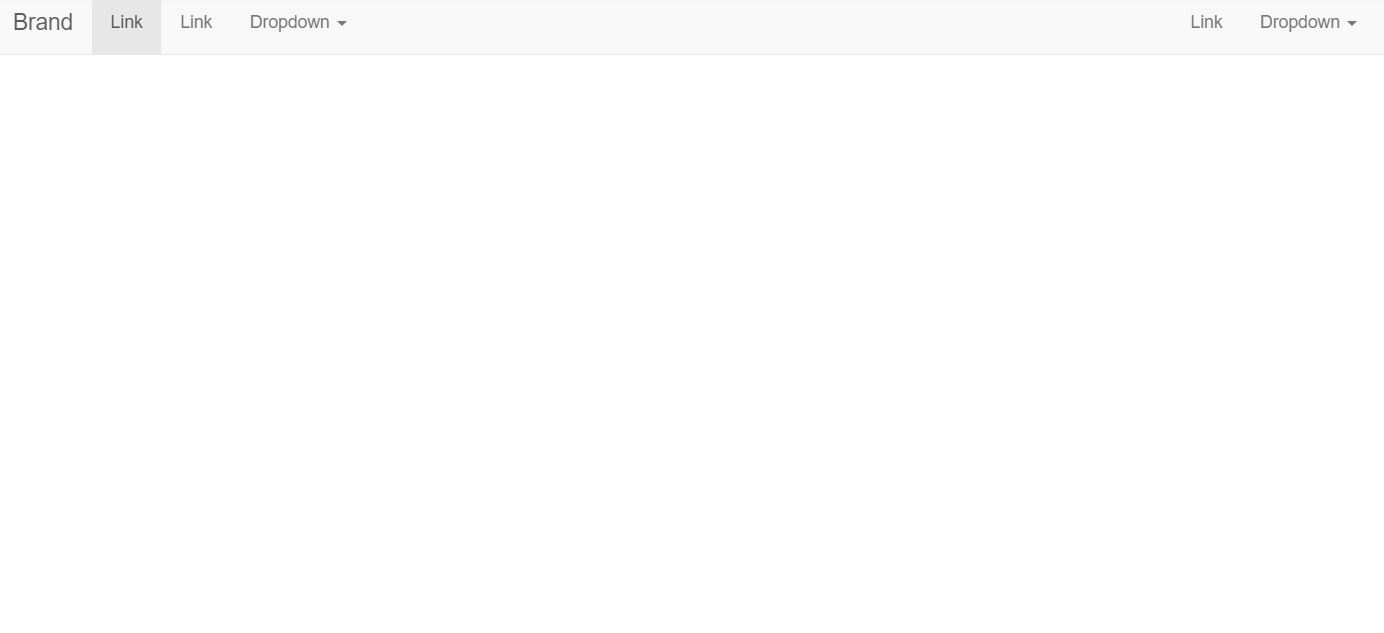The image presents a minimalistic, light grey navigation bar situated at the top. The bar is segmented into distinct sections: a brand link area, followed by a standard link, a drop-down menu, another standard link, and a second drop-down menu. Each section is clearly demarcated, with the "brand link" portion highlighted in a slightly darker grey. The design is simplistic and devoid of any additional images or embellishments. There are no background elements or subtle details to note. The overall aesthetic is clean and straightforward, focusing solely on the functionality of the navigation links and drop-down menus. This unadorned style ensures that the attention remains on the clickable options, making it an easy-to-understand interface.